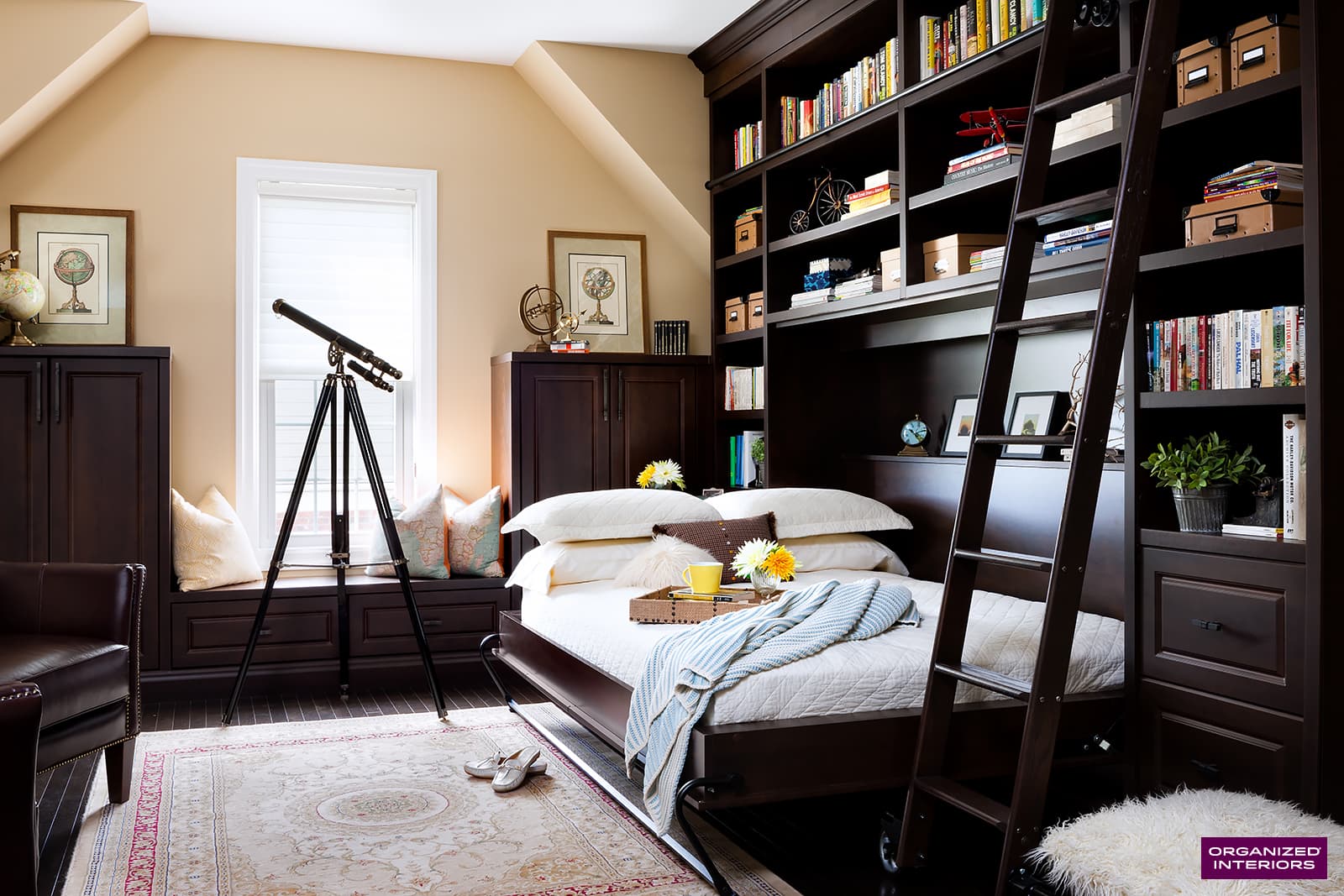The picture features a cozy, well-organized bedroom adorned in predominantly dark colors, almost black, including the bed frame, cabinets, bookshelves, and shelf unit. The centerpiece is a Murphy bed with a light blue blanket, which folds up into a cabinet surrounded by shelves filled with many books. Adjacent to the bed on the right side is a small ladder, used to access the upper levels of the bookshelf. A dark brown chair sits to the left of the bed, separated by an area rug that also has two pairs of shoes.

The room's ceiling is white, complemented by slightly peachish beige walls. In front of the window, a telescope perched on a matching dark brown shelf invites stargazing. The window is flanked by two dressers, also in dark brown. On top of a cabinet to the left, a globe and a painting of a globe add an academic touch. The bed is adorned with a small table holding a yellow coffee mug, some white and red flowers, and three pillows are placed on a nearby stoop. This carefully curated space is both functional and peaceful, perfect for relaxing or engaging in a bit of late-night reading or stargazing.